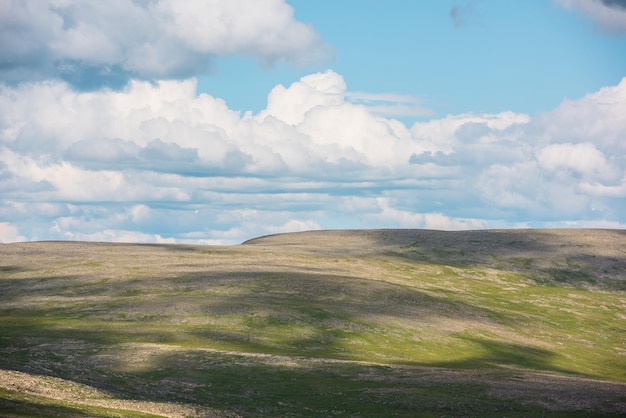This image captures an expansive, open landscape that appears to be taken from an aerial view, showcasing a slightly rolling, grassy hill with patches of green interspersed with areas of gray or brown, revealing sand-colored dirt beneath the sparse vegetation. The land gently slopes near the horizon, contributing to the serene prairie setting. Above, the sky varies from a baby blue to a medium blue, dotted with diverse clouds that become more concentrated towards the horizon. Some clouds are dark, casting shadows over the fields below, while others are white and billowing, creating a tranquil, picturesque scene devoid of any human presence.